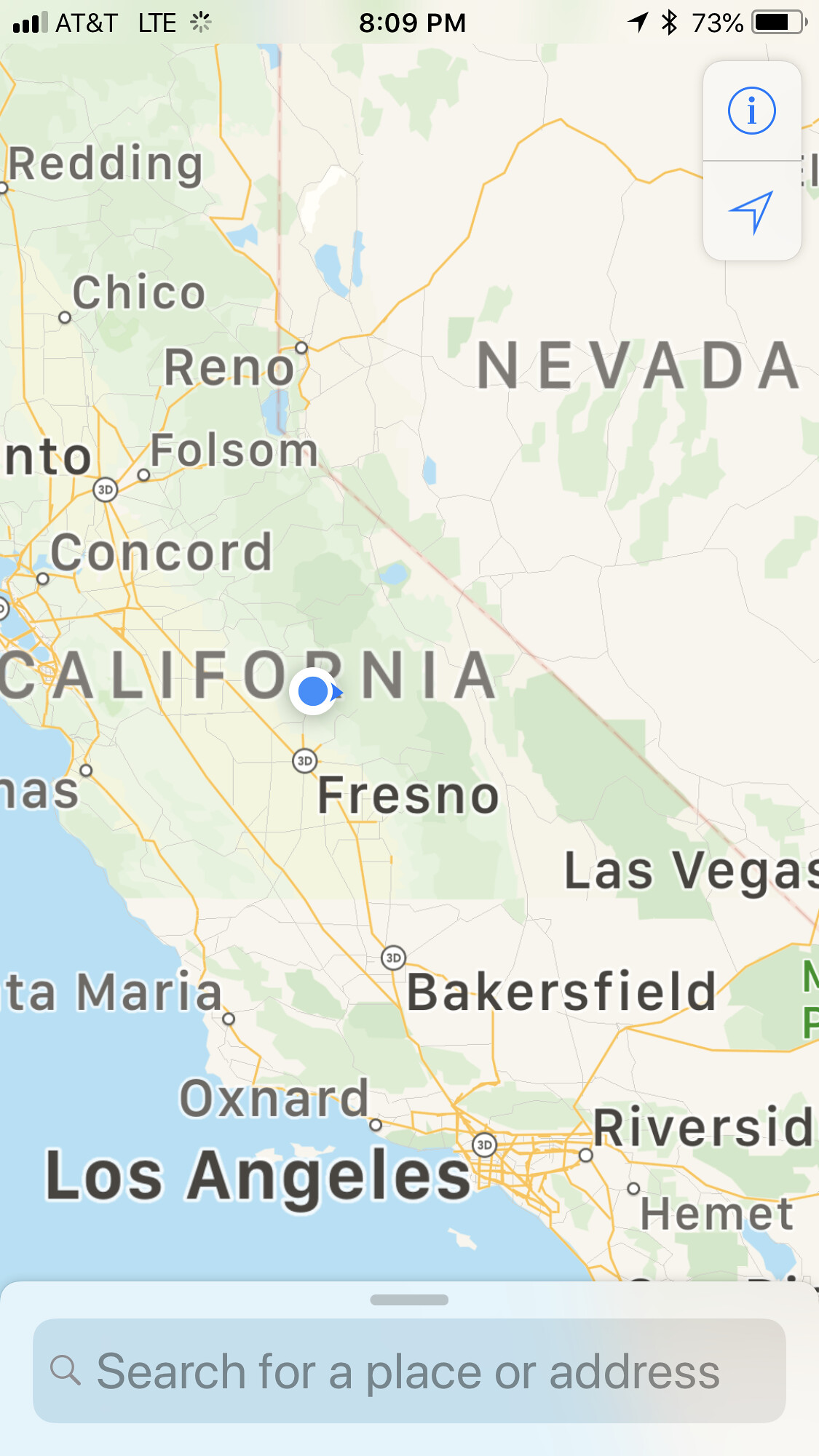This photograph depicts a digital map displayed on a mobile device, likely a smartphone or tablet. The map features a segment of the western United States, specifically highlighting areas of California and Nevada. The visible range extends from south of Los Angeles up to north of Redding. A distinct blue dot is positioned just north of Fresno, pinpointing the current location of the user accessing the map. This blue dot is a common feature in Google Maps, indicating the user’s real-time location, which, in this case, places them at the 'R' in "California" on the map. Above, a small portion of the map includes the city of Sacramento. Additionally, at the bottom of the screen, there is a search box that reads "Search for a place or address." Other on-screen details reveal that the device is connected to an AT&T LTE network, it is currently between 8 and 9 p.m., and the battery level is at 73%. The overall display suggests active usage of Google Maps for navigation or location search.